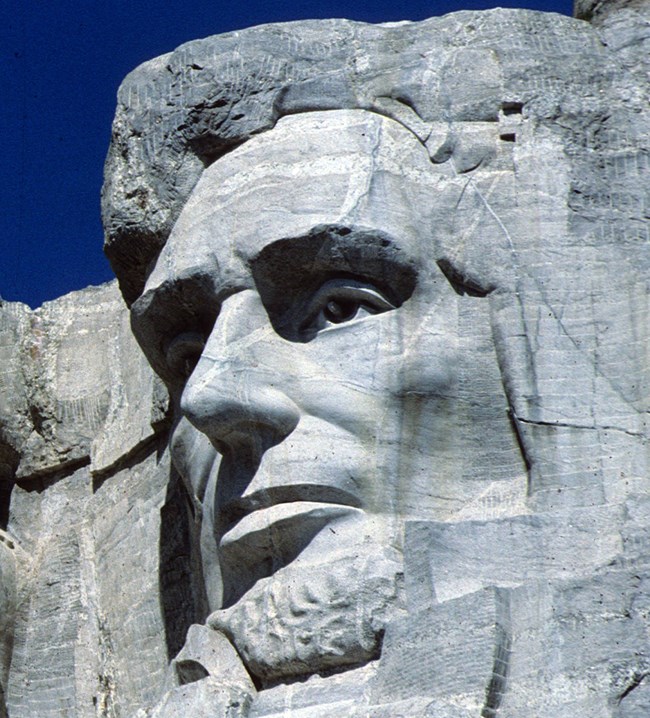The image is a vertically oriented, close-up photograph focusing exclusively on the Abraham Lincoln section of Mount Rushmore. The detailed carving of Lincoln's face is prominently displayed, capturing his serious expression and the distinctive features of his visage. The left side of his face is prominent, revealing the intricate details like his hooded eyebrows, pronounced nose, chiseled cheeks, and short, curly beard. Shadows accentuate the depth around his eye area and the cheek, where there is also a visible crack. The left side of the image is also shadowed. The rock is naturally gray, adding to the solemn and imposing presence of Lincoln’s face. In the top right corner, a sliver of the dark but bright blue skyline is visible, providing a stark contrast to the gray stone. Minimal surrounding mountain is visible to the left of Lincoln’s face, emphasizing the isolated focus on his monument.